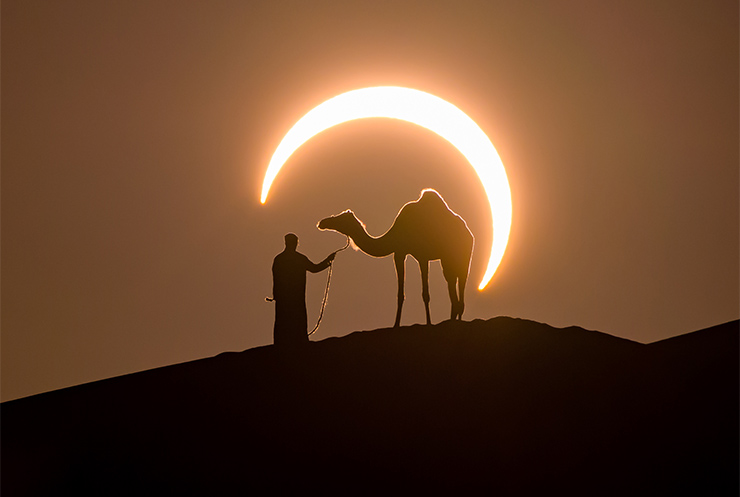In this professional photograph, a captivating solar eclipse bathes the sky in ethereal shades of black and orange. The crescent sun, partially obscured by the moon, casts dramatic shadows over a serene desert scene. Perched atop a rolling sand dune, a majestic camel with a single hump stands silhouetted against the luminous sky. Beside the camel, a man dressed in a long black cloak holds a rope, guiding the animal. He stands close, with the rope draped loosely in his left hand. The intricately framed crescent sun arches elegantly from the left, almost above the man’s head, to the right, highlighting the unique position of this celestial event and casting an otherworldly glow on the figures below.